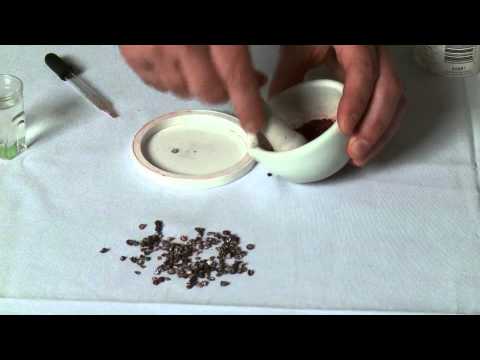The photograph depicts a detailed scene of someone, likely a man, preparing a substance that could be medicinal or a spice mixture. The scene is framed by thick black borders at the top and bottom, but not on the sides. Set against a white tablecloth, the foreground features scattered black specks, perhaps peppercorns or flax seeds. Central to the image, we see male hands holding a small white ceramic mortar and pestle, actively grinding the contents within the bowl. To the left of the hands (right side from the user's perspective), there's an eyedropper and next to it, a small glass bottle containing a liquid, which could be water, oil, or glycerin. A possible additional container can be glimpsed in the upper right corner. This tableau, marked by a careful and intentional arrangement of objects, suggests a focused process of creating something, potentially medicinal due to the associated eyedropper and liquid container.